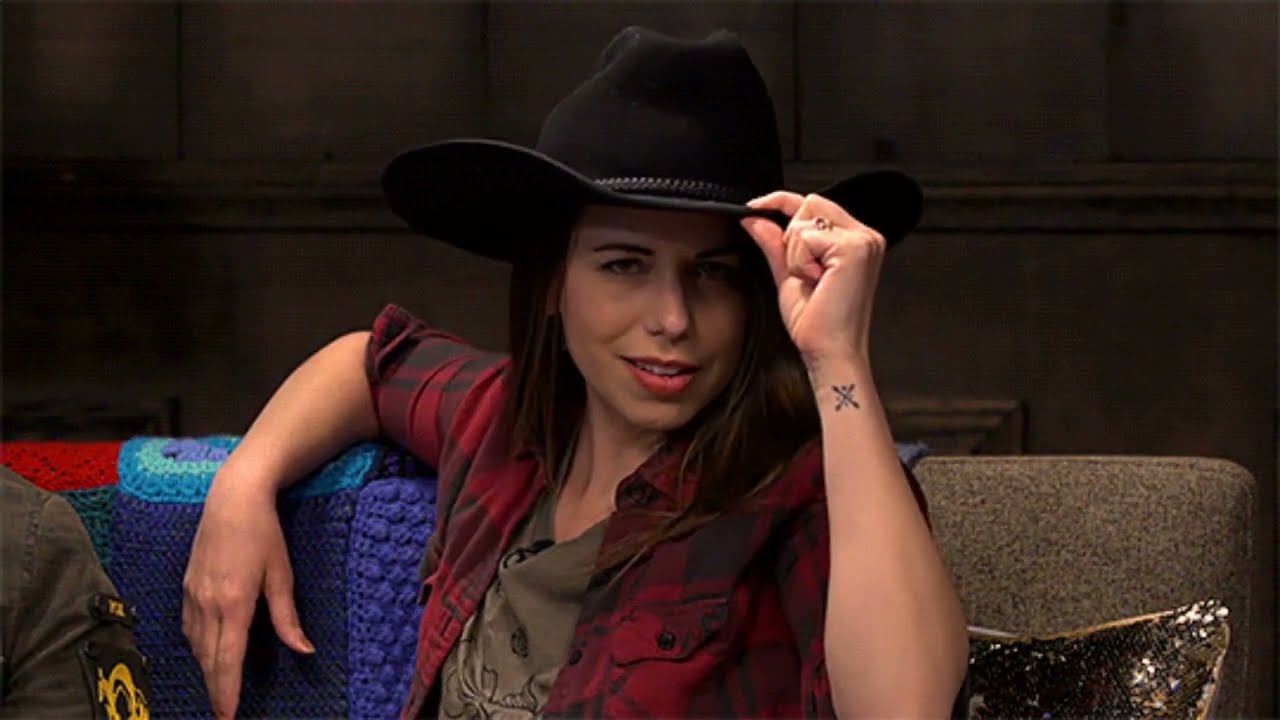In this wide rectangular image, a light-skinned woman is sitting on a gray couch with her right arm draped over the back and her left hand tipping a black cowboy hat adorned with a leather band. She has a subtle grin and dark hair falling over her shoulders. She wears a black and red plaid shirt with an open front, revealing a camo green t-shirt underneath. Both shirts have visible pockets. On her right wrist, a small cross tattoo is visible. Behind her, a quilt with crocheted patches in blue and multicolored hues is draped over the couch. To her left, a hint of another person wearing what appears to be a military-type jacket with a patch on the arm can be seen in the bottom left corner of the photo. The background consists of large, dark brown wall panels with horizontal molding. There is also a gold sequin pillow leaning in the corner of the couch.